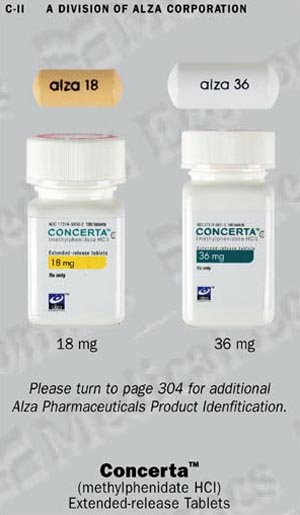In this image, two prescription pill bottles are displayed side-by-side, showcasing a comparison between two different dosages of the medication Concerta. Both bottles are predominantly white, featuring white labels and white lids, and are centrally positioned against a plain background.

The bottle on the left is slightly shorter in height but compensates with a taller white lid. The label on this bottle reads "Concerta" in green at the top, followed by "18 milligrams" highlighted in yellow. Below this, the label specifies "prescription only" and features an emblem resembling a white spiral on a blue background. The 18 mg dosage is reiterated beneath the emblem. Above the label's text, there is an illustration of the actual pill: a squat, short, beige-colored tablet inscribed with "18" on its side.

The bottle on the right, while taller, has a shorter lid. Its label mirrors the design of the first but indicates a higher dosage. "Concerta" is printed in green at the top, with "36 milligrams" highlighted in green instead of yellow. The blue spiral emblem appears here as well, with "36 milligrams" mentioned below it. At the very top, the label notes the manufacturer as a division of some corporation, abbreviated as "CI." The label instructs viewers to see pages three or four for additional product identification details related to Concerta, and includes the scientific name of the medication followed by "extended release tablets" in parentheses.

Both bottles are centered in the image, with clear visibility of their detailed labels and the distinctive markings differentiating the dosages.